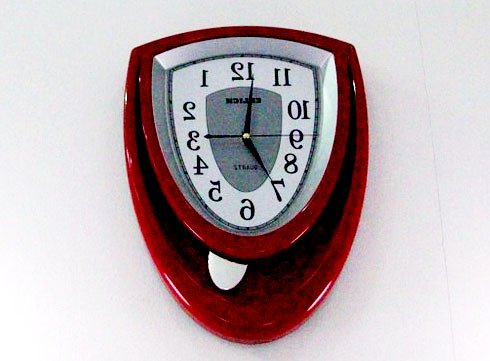This is an image of a uniquely designed wall clock, crafted from red plastic and shaped reminiscent of a knight's shield. The clock's face is set against a solid white background and features an interior white space with black numbers and hands. The numbers are presented in a reversed and flipped format, making the clock a mirror image of a traditional timepiece. At the top, the number 2 appears backwards, followed in descending order around the dial with the numbers continuing in mirrored fashion: 1 in reverse, then 11, 10, and so on, with 3 located where 9 would typically be. The clock hands are also black, with thick hands indicating 12 and 7, and thinner hands pointing at 9 and 3. Below the main body of the clock, the red plastic extends further, creating a dripping effect that enhances its unconventional appearance. This clock is mounted on a wall that appears to have paneled structures, contributing a subtle architectural interest to the scene.